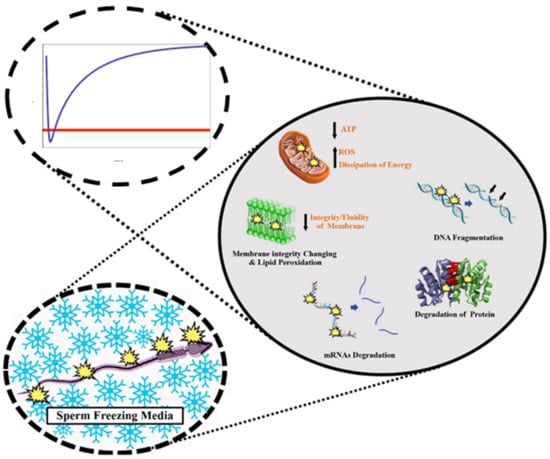The illustration resembles a medical or genetics textbook diagram featuring interconnected ovals, depicting various biological processes related to sperm preservation and cellular metabolism. The image consists of three ovals:

1. **Top-left Oval**: This oval has a dashed outline and contains a graph. The graph is represented by a blue checkmark-like line that starts high on the y-axis, descends sharply, and then curves upward to the upper right. A horizontal red line denotes the x-axis. This section likely represents a biological measurement or reaction over time.
 
2. **Bottom-left Oval**: Also with a dashed outline, this oval is labeled "sperm freezing media." Inside, it features an illustration of a purple sperm surrounded by yellow flashes, set against a background of ice crystal-like snowflakes, symbolizing the freezing process and its effects.

3. **Right Oval**: The largest oval with a solid black outline details several cellular processes. It highlights the dissipation of energy (ATP), DNA fragmentation, protein degradation, mRNA degradation, and changes in membrane integrity. Visuals include DNA strands, cellular molecules, and degradation pathways, all rendered in various colors to indicate different stages and components of cellular metabolism.

Dots in a straight line connect the ovals, emphasizing their relation to one another within the context of the diagram.